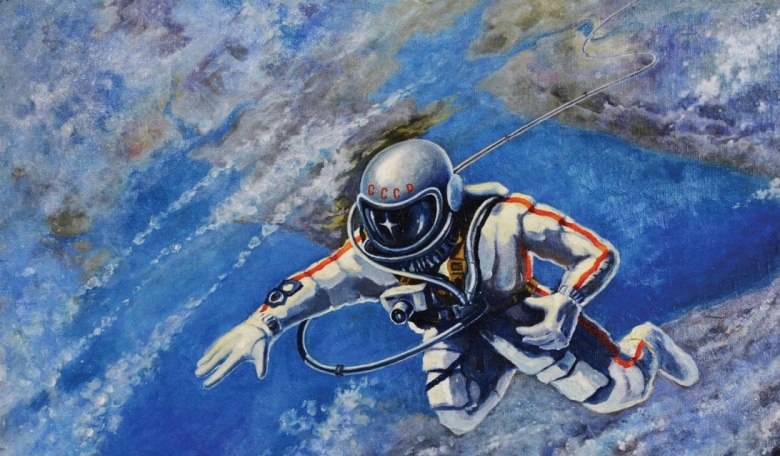The image is a rectangular, cartoon-style drawing measuring approximately six inches wide and three inches tall. It depicts a Russian cosmonaut floating in space, with the Earth visible below. The cosmonaut wears a silver helmet marked with the red letters "CCCP" and a white spacesuit adorned with an orange stripe running down the sleeves and the sides of the legs. His right arm extends outward to the left, while his left arm is bent at the elbow, and his legs are also bent at the knees. A tether line, originating from the upper right, zigzags its way to connect with the cosmonaut. Suspended around his neck by a leather strap is a camera, floating in front of him. The Earth beneath showcases vast blue oceans with scattered landmasses in browns and greens, and an overlay of white and gray clouds, resembling raindrops scattered across the canvas. The cosmonaut occupies the majority of the bottom right corner, facing the left, and stands out vividly against the backdrop of the planet below.